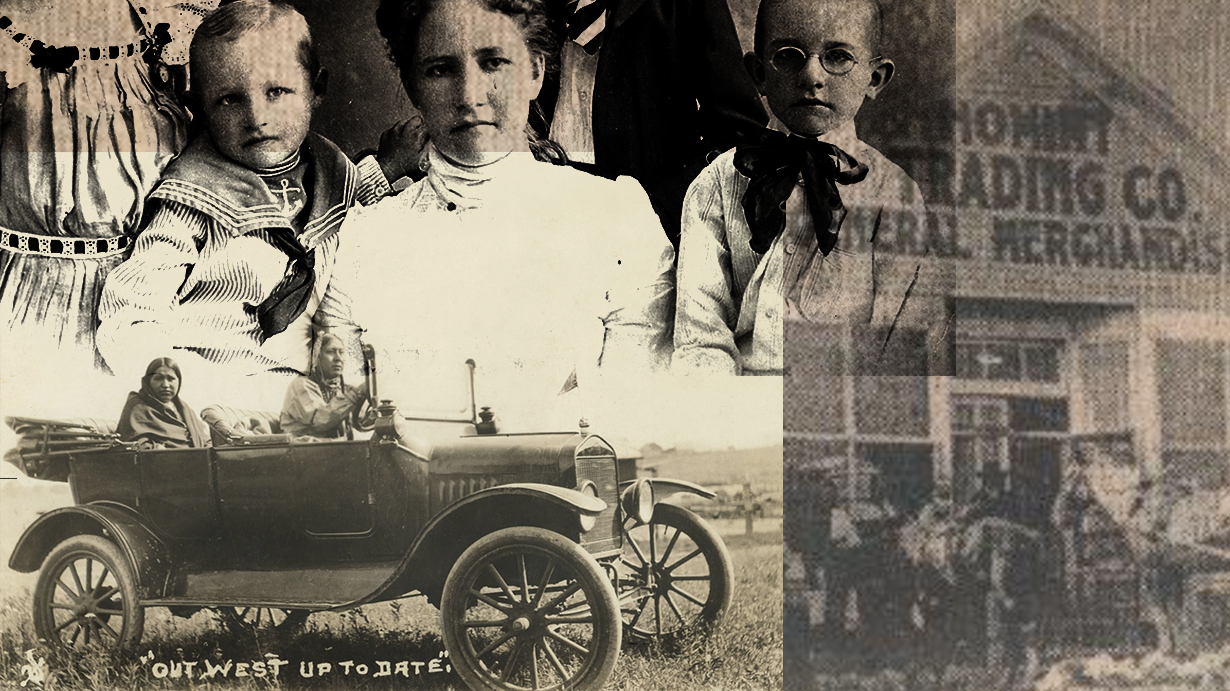This sepia-toned composite image features three overlapping, early 20th-century photographs, each offering a unique glimpse into historic American life. 

In the bottom left section, a vintage car resembling a Model T is occupied by a Native American man and woman; the man, in the front seat, dons a small headdress, while the woman, in the back, wraps herself in a traditional blanket. The handwritten caption beneath this scene reads, "Out West Up-to-Date," suggesting a blend of tradition and modernity.

Above, in the upper left, a woman with her hair up stands alongside two children. The boy on the right sports slick-backed hair, glasses, a button-up shirt, and a large bow tie, while the child on the left, possibly in a sailor suit with an anchor emblem, appears next to an old-fashioned skirt or dress. The vignette captures a family moment frozen in time.

To the right, the image of a building marked "Hominy Trading Co. General Merchandise" stands out, suggesting it is a local general store. The scene is grainy, but it depicts individuals gathered in front, possibly customers or townspeople. A man in a hat is faintly discernible, and the setting implies a bustling focal point of a past community.

Together, these interconnected images paint a richly detailed portrait of early 20th-century America, juxtaposing elements of Native American culture, everyday family life, and the hub of small-town commerce.